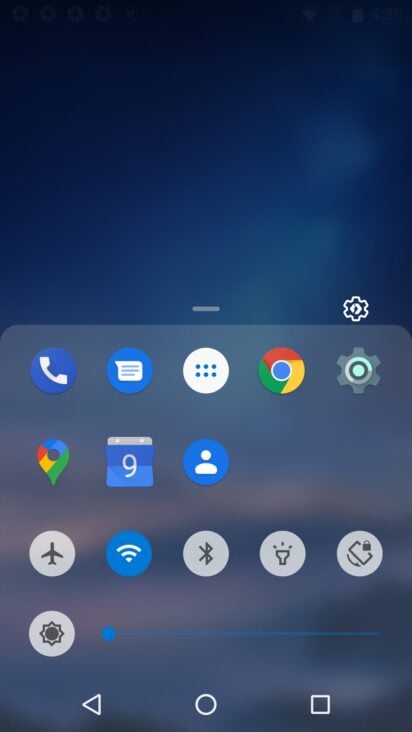This image is a detailed screenshot of an Android smartphone's home screen with a slightly unconventional layout. The navigation bar at the bottom displays the familiar icons: a left-pointing arrow for 'back,' a circle for 'home,' and a square for 'recent apps,' confirming the Android operating system.

Dominating the center of the screen is a semi-transparent window that appears to be an app drawer or a quick settings panel, which can be adjusted in size by pulling a small handle. This handle sits below a central settings cogwheel icon, which is prominently placed, slightly above the middle of the screen.

The background of the screen is a dark blue, resembling the Milky Way, with darker edges and a lighter center, adding a galactic feel. Hints of orange or yellow are visible through the translucent window, somewhat evocative of a cityscape illuminated across a river at night, although it remains abstract.

Within the pulled-up window, a variety of icons are organized:

- **Top row (application shortcuts):**
  - Phone icon
  - Messages icon
  - An icon with six dots for accessing further options or apps
  - Google Chrome icon
  - Another settings cogwheel icon

- **Second row (additional application shortcuts):**
  - Google Maps icon
  - Calendar icon
  - Contacts icon

- **Bottom row (quick settings):**
  - Airplane mode icon (not highlighted)
  - Wi-Fi icon (highlighted in blue, indicating it’s active)
  - Bluetooth icon (not highlighted, indicating it’s off)
  - Flashlight icon
  - Screen rotation lock icon
  - Another settings icon, potentially for display settings, with a blue-highlighted slider set to minimum brightness.

This comprehensive screenshot provides an insightful glimpse into the unique customization and organizational structure of this Android device’s user interface.